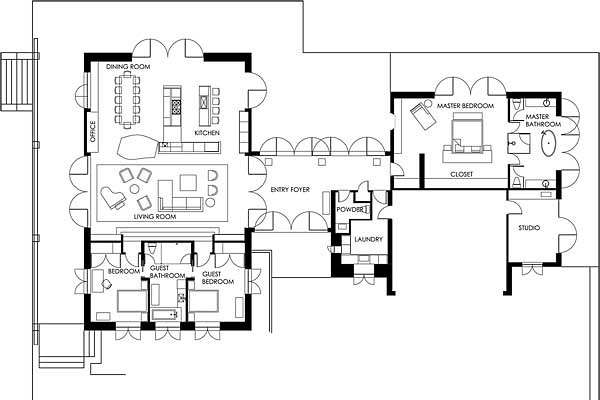This black and white overhead drawing depicts a detailed floor plan of a home, though it's unclear if it's a single-family house or an apartment. The layout starts with stairs outside the structure leading to both a front entrance on the left and a possible side or private entrance at the bottom. Entering through the side entrance, you immediately encounter a bedroom, identifiable by the presence of windows next to the stairs. Adjacent to this bedroom, to the right, is a guest bathroom followed by a guest bedroom.

From this hallway, moving upward leads to the living room, which is elegantly furnished with a baby grand piano, a sectional sofa, sitting chairs, and a coffee table. Continuing further up the layout, you find a modestly-sized office. Adjacent to the office, heading further up, is the dining room. Walking through the dining room brings you to the kitchen, equipped with a six-burner stovetop.

Exiting the kitchen to the right, you find the entry foyer. To the side of the foyer are a powder room and a laundry room. Proceeding further through the foyer leads to the master bedroom, which features a king-size bed. This master suite includes a master bath, a spacious closet, and an additional studio area.